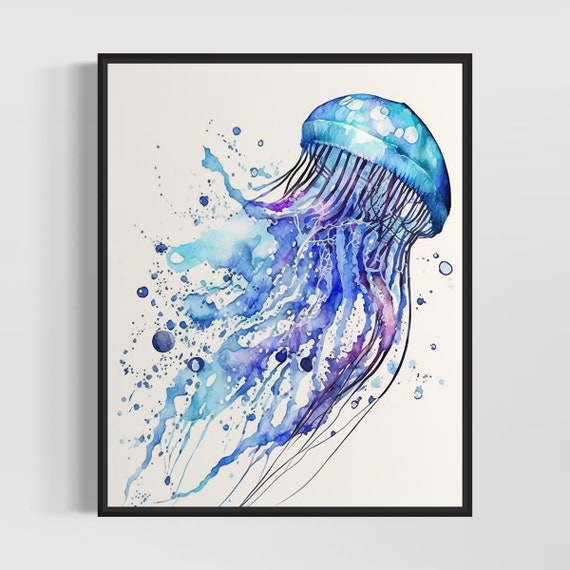The artwork presents an abstract depiction of a jellyfish, framed by a simple, thin black frame and set against a pale blue wall. The piece appears to be painted with watercolors, predominantly featuring shades of blue, purple, and black with touches of green. The jellyfish occupies the upper right corner of the painting, with its cap and tentacles extending downward. The tentacles vary in thickness and color, some being black while others are blue, creating a dynamic motion effect. Surrounding the jellyfish are bubbles, enhancing the impression of an underwater scene. The background of the artwork is white, allowing the vivid colors of the jellyfish and the abstract splatters of paint to stand out. The painting balances realistic elements with an expressionistic style, offering a visually compelling and ethereal underwater landscape.